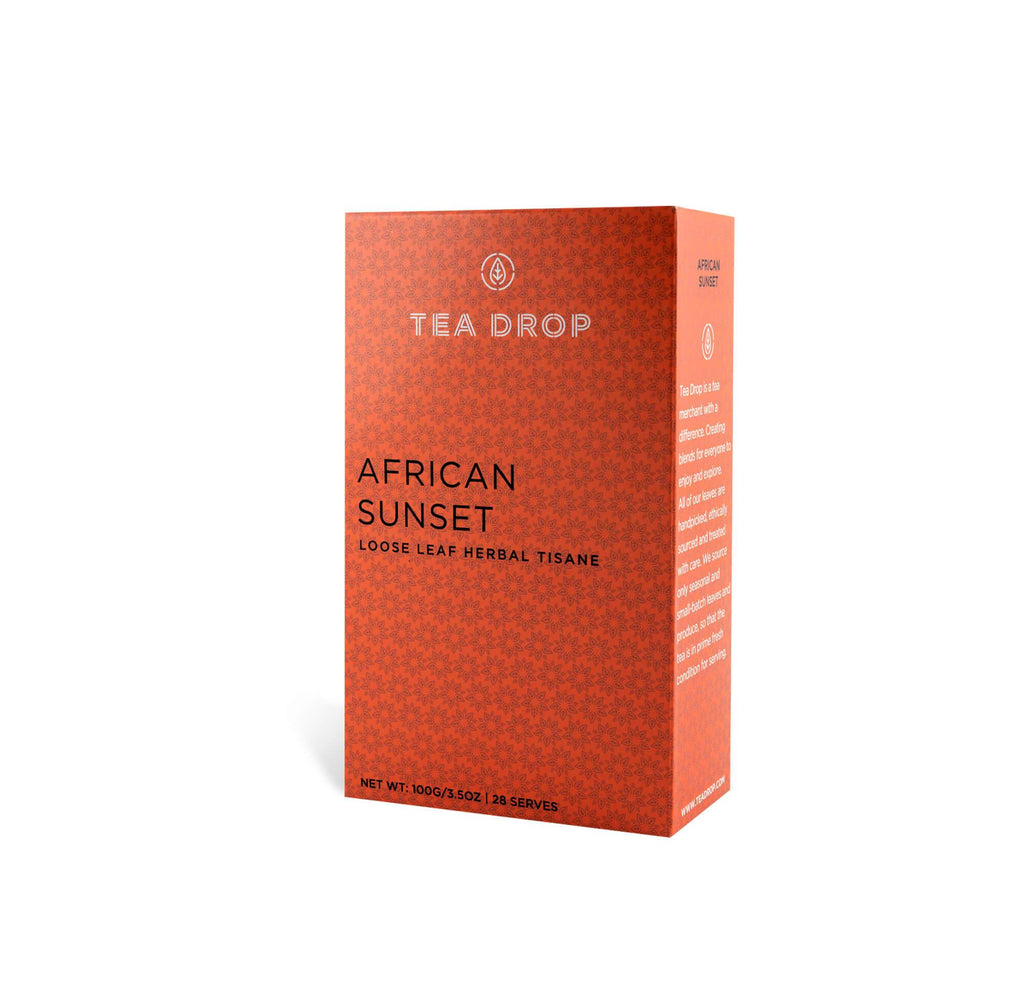This is an image of a vertically oriented, book-sized rectangular box of tea named "Tea Drop." The box is vibrant orange, adorned with a light brown floral pattern that lends a delicate touch to the design. Centered prominently on the front, at the top, is the Tea Drop emblem followed by the brand name "Tea Drop" in bold, bright white capital letters. Midway down the front, in contrasting black text, the label reads "African Sunset," and further specifies "loose leaf herbal tisane" beneath it. At the very bottom, the packaging details the net weight as 3.5 ounces (100 grams) and mentions that it serves 28. The box's right side also has inscriptions, likely a description of the tea, though they are not clearly legible in the image. The overall appearance of the box is centered and visually appealing, with detailed information and elegant design elements.